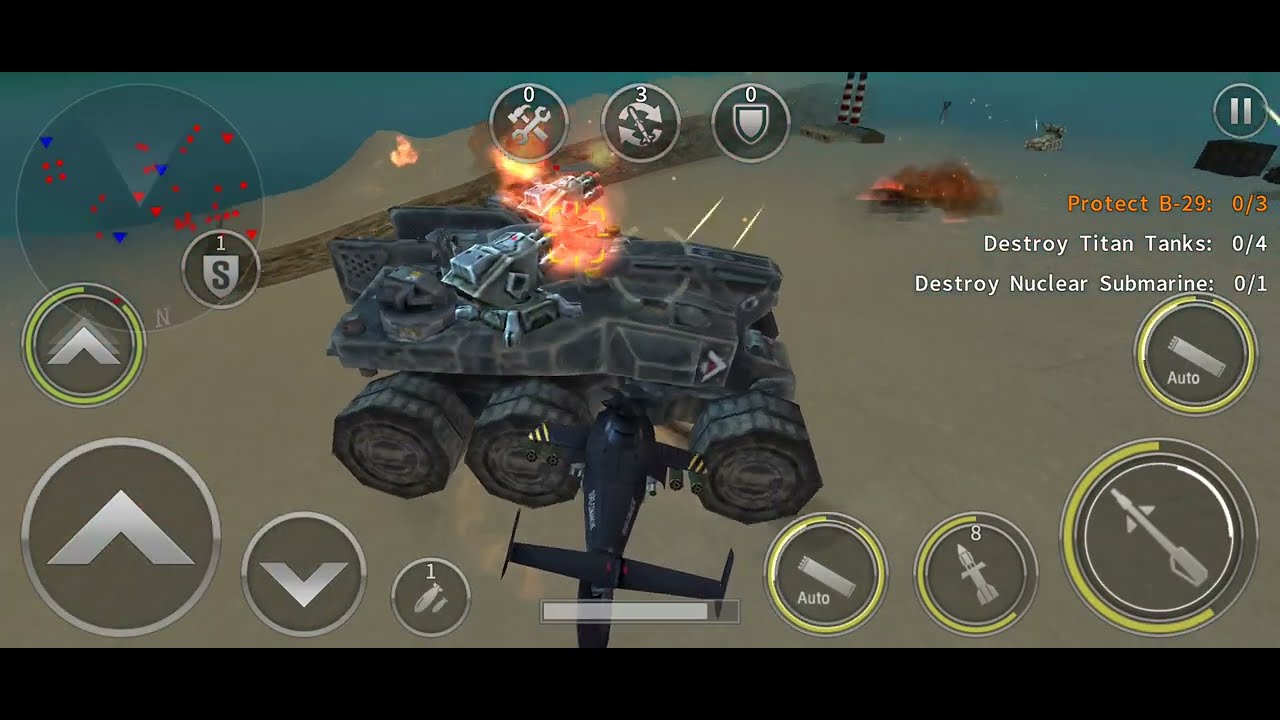This image is a detailed screen capture from a video game, featuring a tense desert combat scene. The landscape orientation is framed by thin black bars at the top and bottom. Dominating the center of the image is a formidable tank mid-fire, launching its cannon towards another vehicle or object in the distant background. This central tank, adorned with camera-like lenses sticking out from its body and extensions on its front wing, is engulfed in fiery explosions above its turret. Visible overhead is a helicopter, adding to the chaos of the battlefield.

Active ammo and visible explosions highlight the intensity of the ongoing battle. The backdrop reveals part of a structure with towering stacks, setting the scene amidst a barren desert terrain. Overlaying the action are various gaming interfaces, including a mini-map positioned in the top left corner.

The game appears paused, with crucial mission objectives prominently displayed. In orange text at the top right corner, it reads: "Protect B-29, 0 out of 3." Below that, white text states: "Destroy Titan Tank, 0 out of 4," followed by "Destroy Nuclear Submarine, 0 out of 1." Additional interface elements, such as weapon symbols and navigational buttons in a chrome design, are scattered along the bottom left and left side, contributing to the intricate HUD of this war-themed video game.